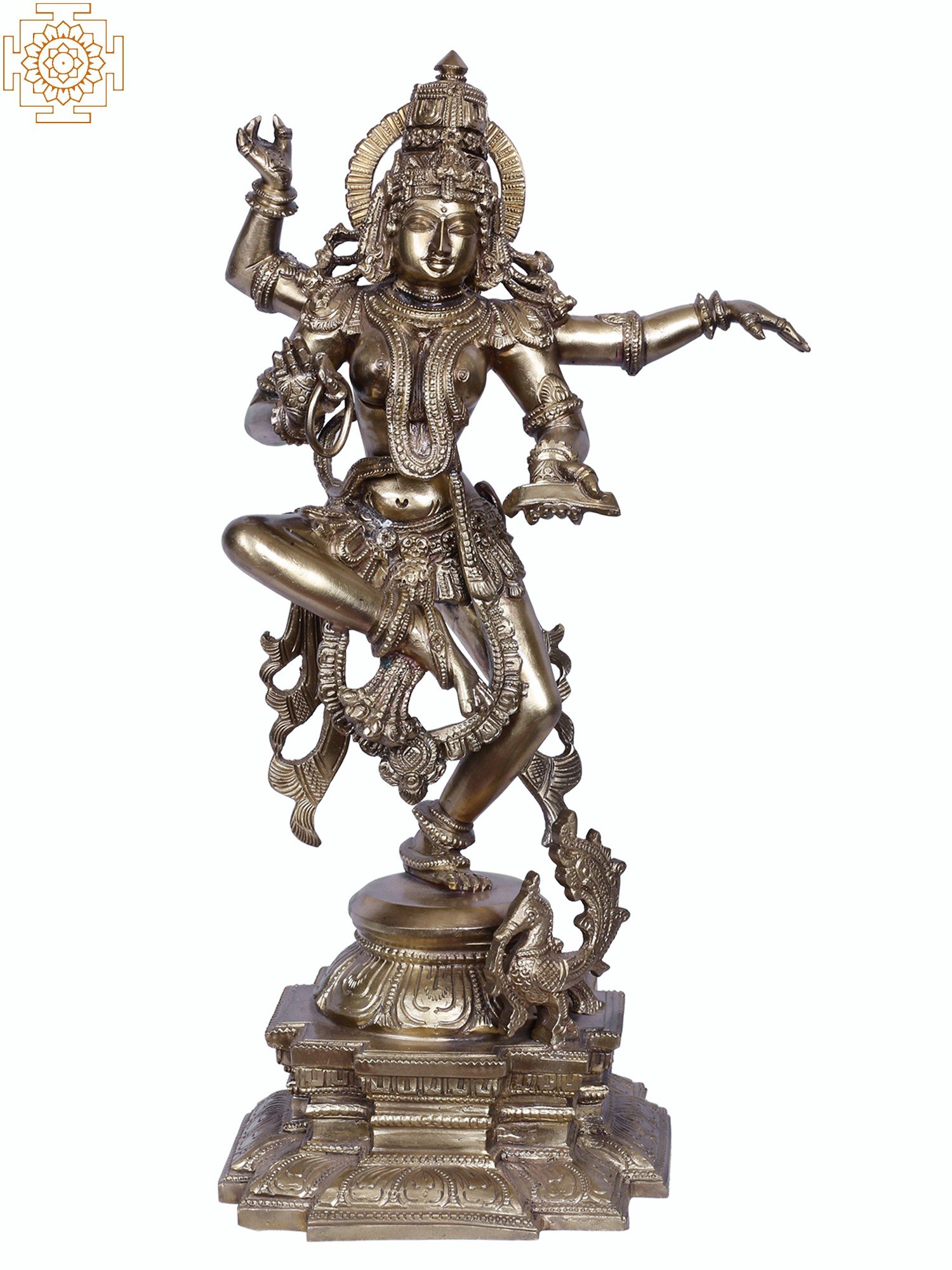This image showcases an intricate bronze or gold-colored statue of a Hindu deity, likely Shiva Nataraja, known for his dynamic dance pose. The deity is depicted with four arms, elegantly posed in a dancing stance with one leg bent at the knee, the foot resting on the opposite thigh, while the other leg is firmly planted on an ornate, multi-layered pedestal. The statue features a detailed headdress topped with a vertical design, encircled by what appears to be a halo behind the head, giving an almost crown-like appearance. Each arm holds significant objects: the top left hand is raised palm up, the top right hand is extended palm downwards, while the lower arms carry distinct items, possibly a ring and a tablet. Additional elements like serpentine ribbons or ropes drape across and downward from the deity's body, adding to the complexity of the sculpture. The background is a plain white, which helps to highlight the rich details of the statue, including an intriguing insignia at the top left of the image.